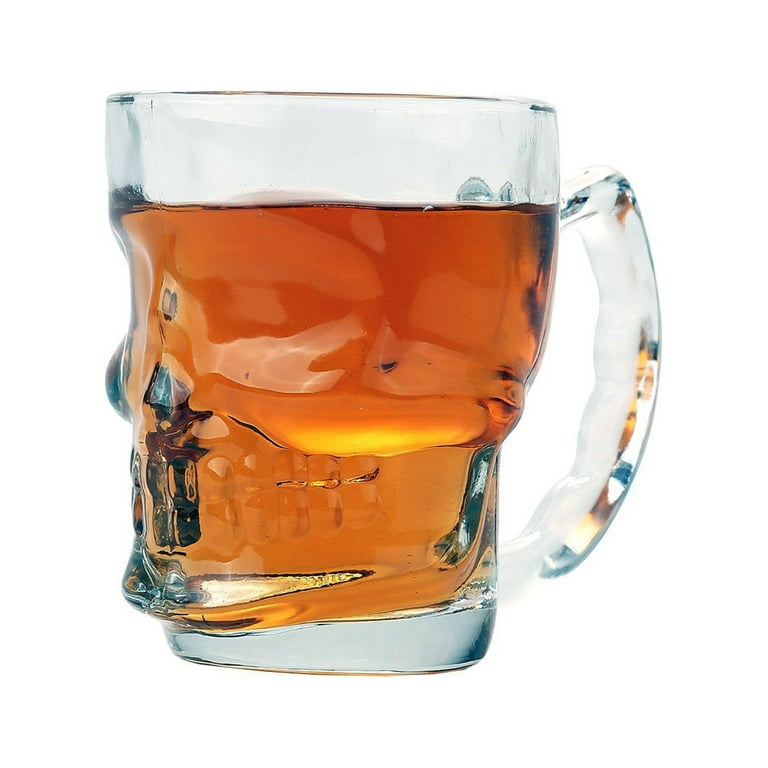This image features a medium-sized, clear glass mug filled with an amber-colored liquid, possibly beer or tea, up to about seven-eighths of its capacity. The mug is oriented to the left, showcasing a distinct and intricately detailed human skull design on its front. The skull design is complete with indentations resembling teeth, eye sockets, and jaw bones, giving it a striking skeletal appearance. The handle, ergonomically designed with indentations and positioned at the back, includes a thumb rest at the top for easy grip. The mug is set against a pure white background, making it suitable for a product photo typically seen in a catalog or product listing. This novelty glass, with its unique skull motif, makes for an interesting gift item.